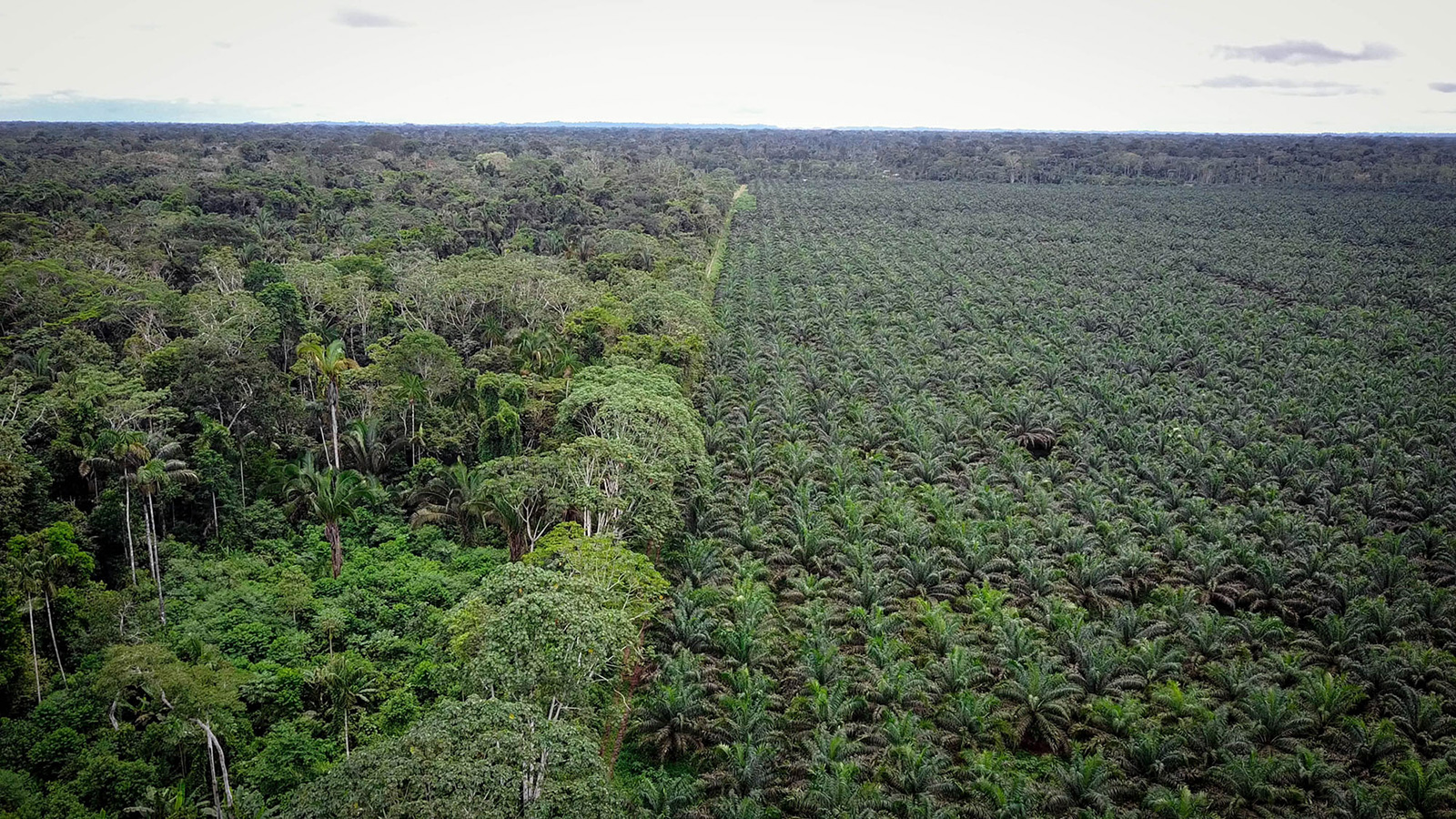This aerial, possibly drone-captured, image presents a striking contrast between two distinct areas of lush greenery in what appears to be a tropical region. On the right-hand side of the image, a neatly parceled rectangular plot is evident, with rows and rows of identical, low-lying plants, possibly small palms or similar foliage with fan-like leaves. Each plant is uniformly placed, suggesting a carefully managed agricultural or orchard area dedicated to a single crop, though the exact type of plant is uncertain. In stark contrast, the left side of the image features a dense, unkempt rainforest or jungle with a rich tapestry of vegetation. The jungle is teeming with a mix of tropical trees, including deciduous and palm trees, growing thickly and chaotically, their branches and leaves intertwining as they stretch towards the sky. The horizon reveals a continuation of this verdant landscape, shrouded under an overcast sky with a hint of white cloud cover. The crafted order of the right-hand plantation sharply contrasts with the wild, natural expanse of the left-hand forest, creating a vivid depiction of human intervention beside untouched nature.